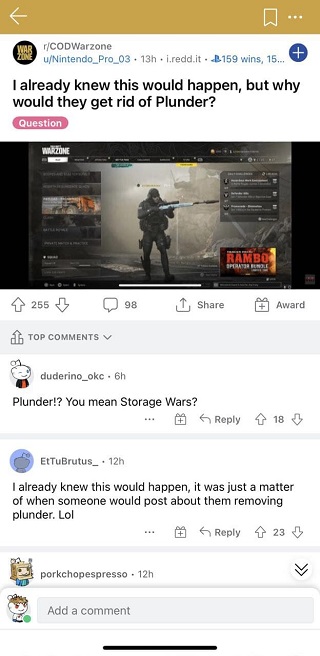**Caption:**

The image depicts a screenshot from a cell phone displaying a Reddit thread in the subreddit r/CODWarzone. The interface features a gold bar at the top with a left-pointing arrow to navigate back, a ribbon-shaped icon to save the thread, and three dots for more options. Below, the Warzone logo is visible, and the post is made by user u/Nintendo_Pro_03, timestamped "13 hours ago," with a partially visible URL ending in "i.redd.it."

The main post title reads, "I already knew this would happen but why would they get rid of Plunder?" This is posed as a question. The attached image is a screenshot from COD Warzone featuring a menu with several selectable options and an image of an in-game soldier holding a long gun.

The post has garnered 255 upvotes and 98 comments. Users have the option to share or award the post. The top comment by duderino_okc, posted six hours ago, reads: "Plunder!? You mean Storage Wars?" The next comment by user ettubrut01, posted twelve hours ago, says, "I already knew this would happen, it was just a matter of when someone would post about them removing Plunder lol." Below this comment, user PorkChopsEspresso also commented twelve hours ago, but their comment is cut off and not fully visible.